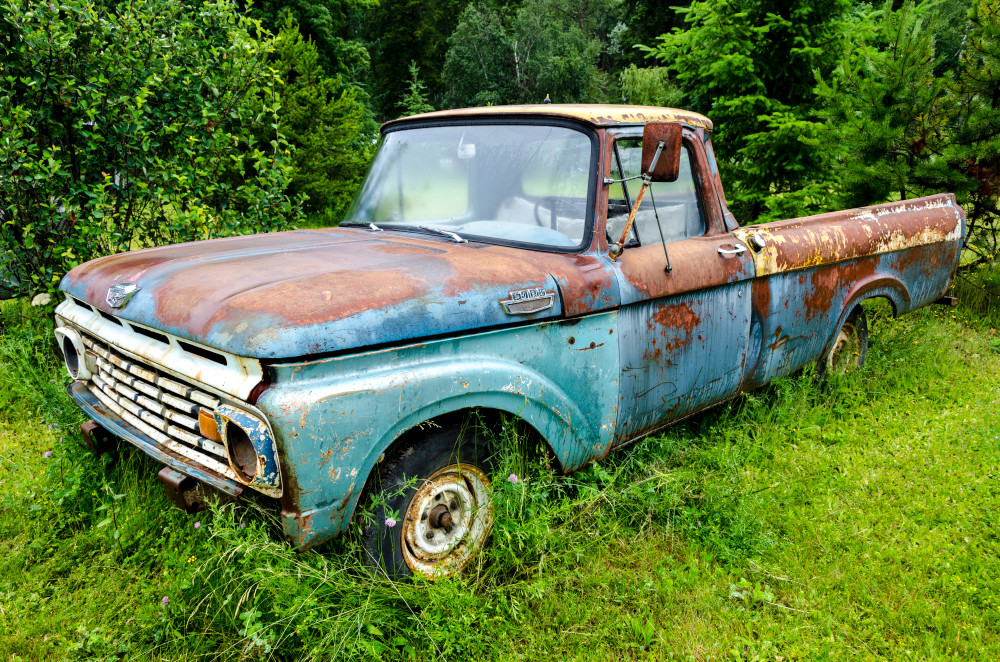The horizontally oriented color photograph captures an abandoned, heavily rusted blue pickup truck sitting in a grassy field amidst a densely wooded area. The vehicle, originally painted a sky blue, shows severe deterioration with significant rust covering the hood, grille, door, and rearview mirror. The grille, once white, still retains some of its original appearance, contrasting the empty headlight sockets. The truck's tires are aged, with rust encircling the rims, and the rear tire appears to be missing or obscured by the grass. Overgrown high grass and trees create a natural frame for the truck, suggesting it has been there for a considerable time. The overall composition, marked by realistic photographic detail, emphasizes the truck's derelict state against the lush, encroaching vegetation.